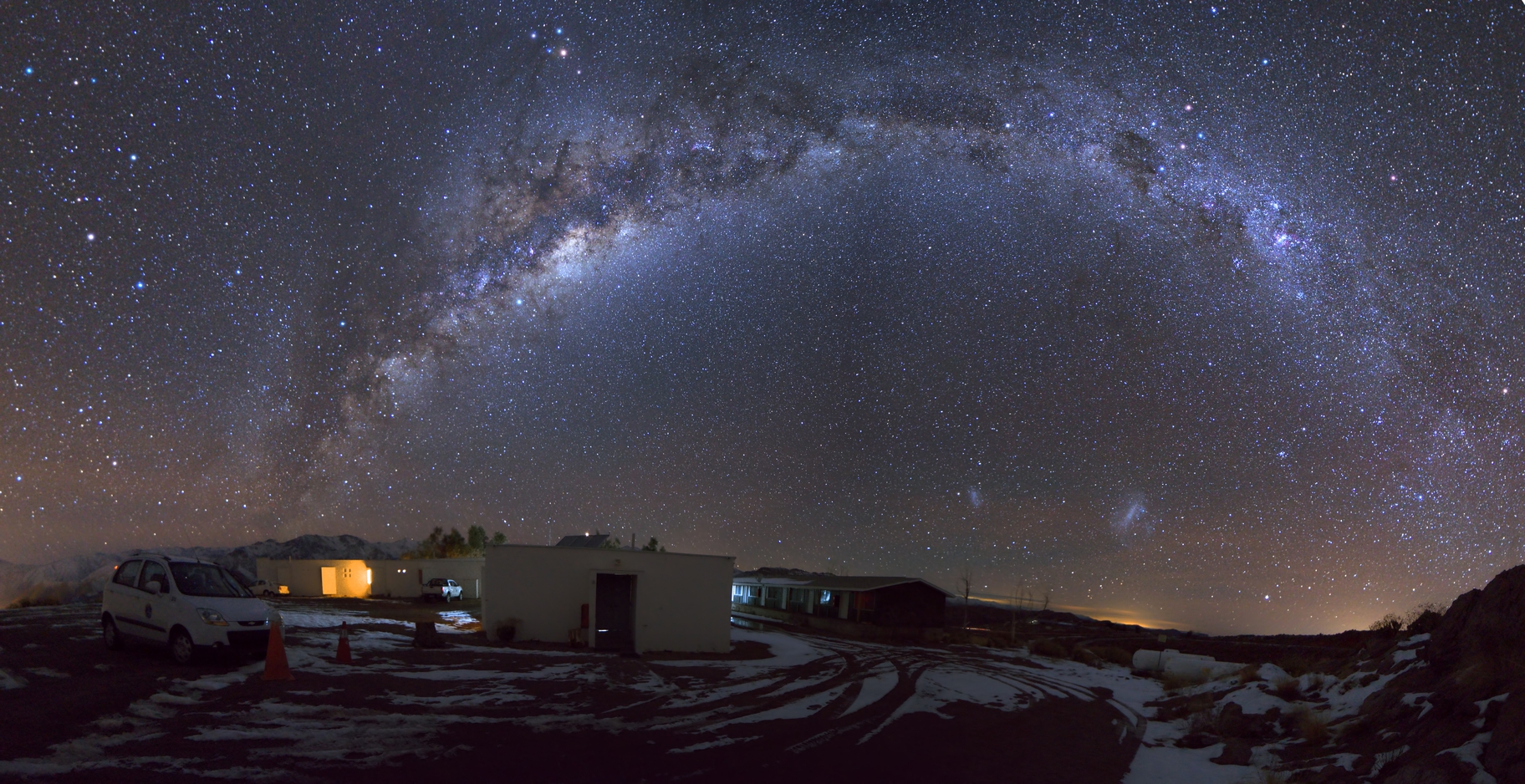This outdoor nighttime photograph captures a snowy and remote location, possibly an area known for stargazing or natural light displays like the Northern Lights. The lower portion of the image shows a snow-covered driveway or parking area dotted with numerous tire tracks. To the left, there are two orange cones and a small white vehicle, presumably an electric hatchback. Centered in the middle of the photograph, there is a well-lit, one-story white building with a door visible, and a truck parked in front of it. On the right side of the image, large white propane tanks can be seen. The upper three-quarters of the photograph showcases a spectacular night sky brimming with stars, including the Milky Way galaxy, which appears as a vibrant, star-filled band arching across the scene. Thin clouds or possibly smoke, forming an arch from the bottom left to the upper right of the photo, add a unique touch to the celestial display. The sky exudes a deep, dark purple hue, enhancing the brilliance of the stars. Despite the absence of people, the illuminated buildings and lights suggest human presence and activity in this serene, snowy landscape.